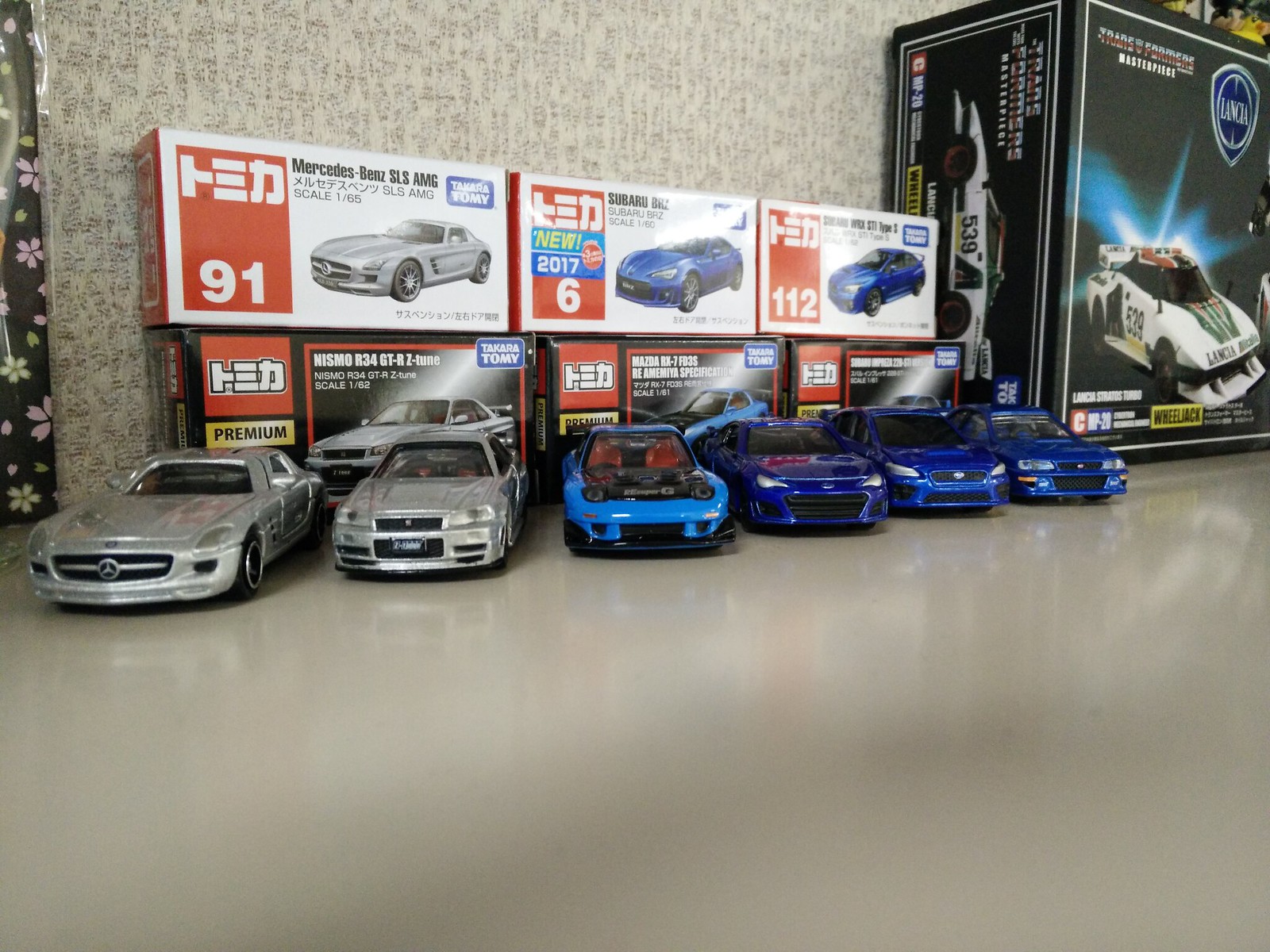The image displays a collection of six model cars meticulously arranged on a reflective, grayish flat surface, adding a shiny effect that captures the reflections of the toys. At the bottom left, two silver cars sit side by side, followed by a blue car with black accents to the right. To the far right, there are three additional blue cars, with one being a darker shade. Behind these models, their packaging boxes are visible. The boxes are primarily black with red squares in the upper left corner, and labeled "premium" in black font outlined in gold. The top row of these boxes includes the numbers 91 on a silver Mercedes-Benz SLS AMG, 6 on a blue Subaru New 2017, and 112 on a final box labeled Hismo R34 GT R2 tuned, which is scaled 1 out of 62. On the far right, a large black box showcases a white car with the Transformers logo and the word LANCIA in white. The background features a gray patterned wall with hints of black, adding depth to the indoor setting.